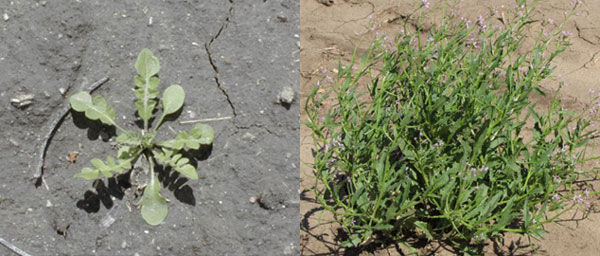The image is a composite of two contrasting sections, each portraying a distinct background and vegetation. On the left side, the background is a dark gray pavement, possibly from a parking lot, with some scattered rocks and pebbles. In the center of this side, a weed with seven leaves, each having multiple sections, grows resiliently. On the right side, the background shifts to light brown, possibly rocky, soil marked by numerous cracks with fewer pebbles. This section features a darker green plant situated closer to the bottom of the image, giving way to a more expansive view of the soil above it. The plant appears more robust and bush-like, suggesting it might be the same weed from the left after receiving water, with small leaves and tiny floral buds, hinting at its growth potential. The overall imagery juxtaposes the harshness of the pavement against the cracked, earthy background, emphasizing the persistence and resilience of plant life in differing environments.